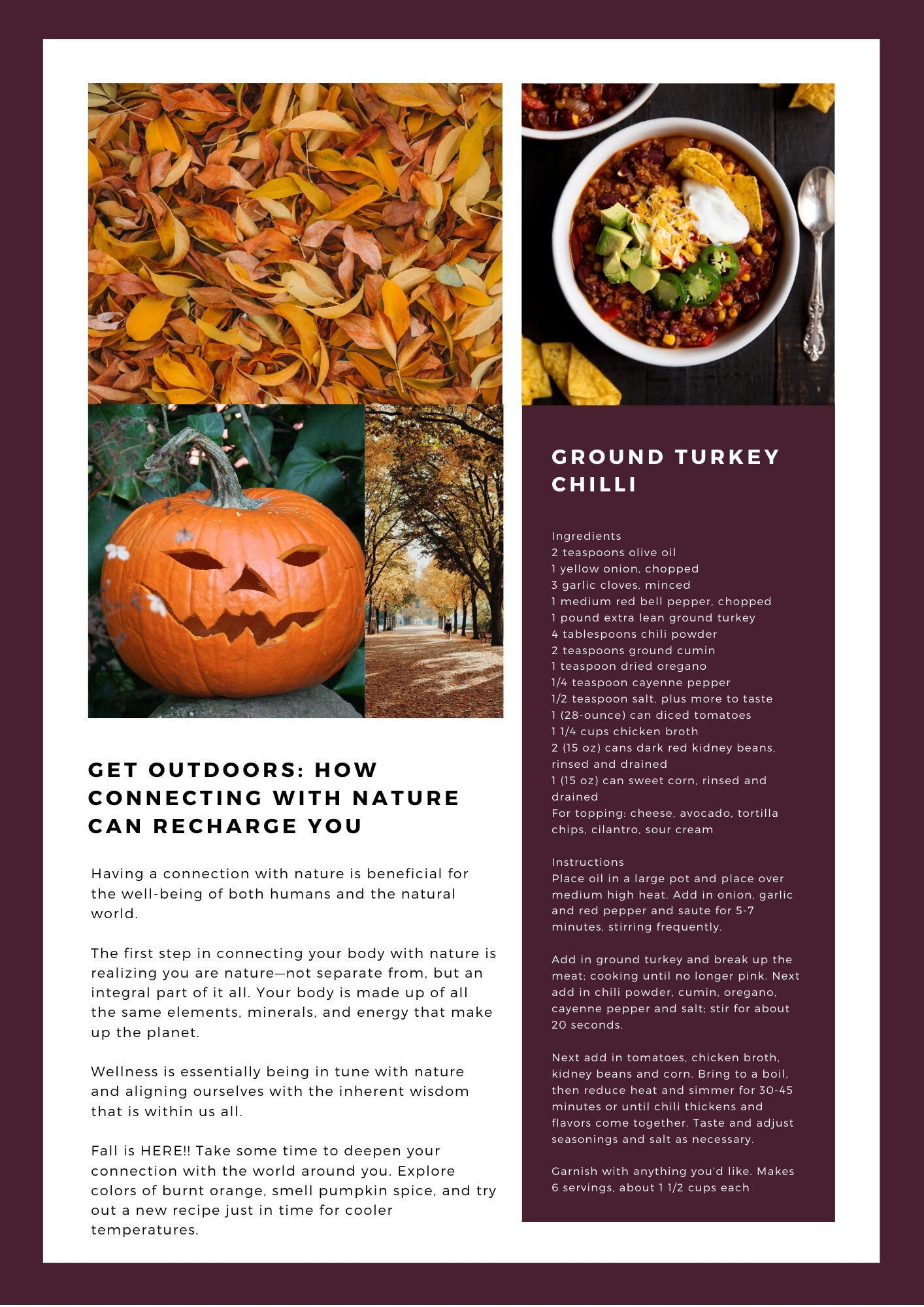The image showcases a maroon screen with a prominent white square in the center displaying a recipe for ground chili. At the top of the visual, vibrant fall leaves cascade, introducing the autumn theme. Below the foliage, a meticulously carved pumpkin adds a festive touch, while on the right, trees adorned with fallen leaves further accentuate the season.

The text within the white square reads: "Get Outdoors: How Connecting with Nature Can Recharge You." It emphasizes the profound benefits of nature for human well-being and environmental harmony. The content advocates for recognizing our intrinsic connection to nature, highlighting that our bodies share the same elements, minerals, and energy as the planet. This mindfulness aligns us with nature's inherent wisdom. 

As autumn arrives, the text urges viewers to immerse themselves in the season – to savor the colors of burnt orange, inhale the scent of pumpkins, and experiment with new recipes suitable for the cooler weather. It then details the ingredients and instructions for preparing a cozy soup and the chili, fostering a deeper connection with the season through culinary exploration.